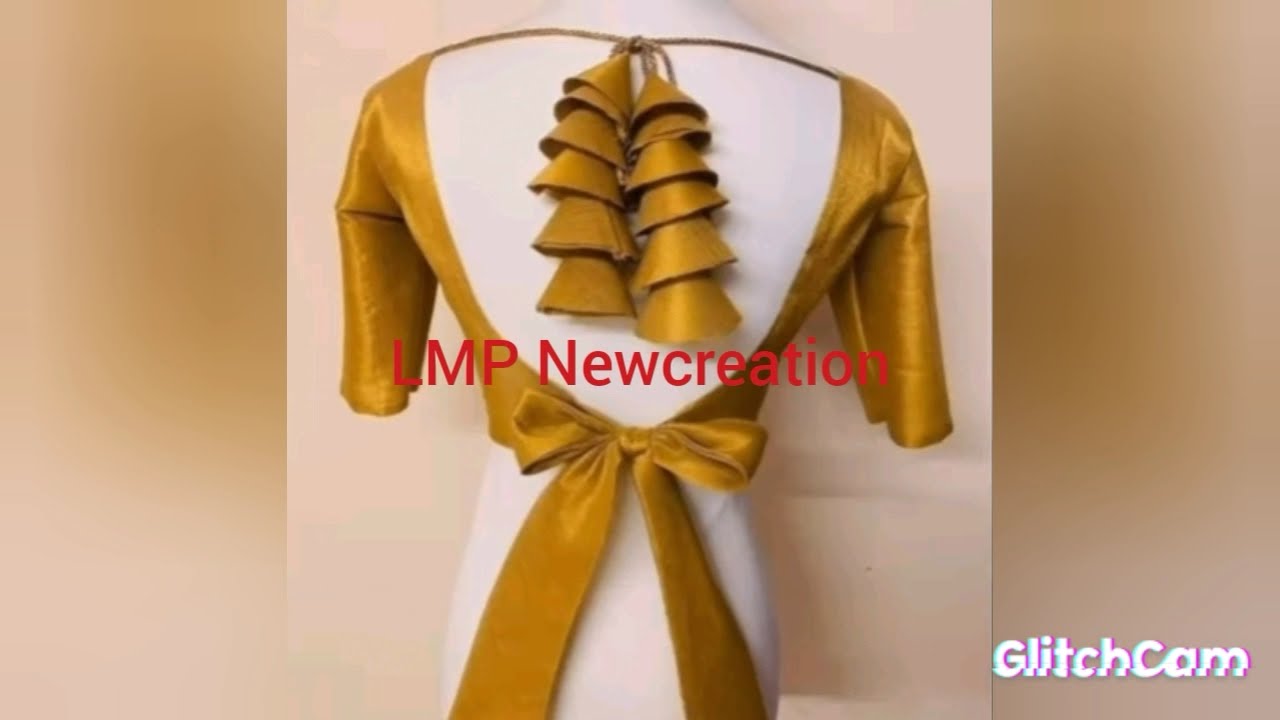The image features a vertical, cell phone-style central picture flanked by thin, tan-colored strips on either side, giving a blurry, cream-brown haze effect. The central focus is on a white mannequin, visible from thighs to shoulders, adorned in a distinctive golden garment. The mannequin appears oriented away from the viewer. The gold top has short sleeves and features a string joining both shoulders at the back, with fabric cascading down in a layered bell fashion. The garment tapers towards the waist, where it's elegantly tied into a gold bow. Above this bow are the red, capitalized letters "LMP New Creation." The borders' unique, blurry tan strips enhance the central image's contrast, and in the bottom right corner of the right border, the words "Glitch Cam" are displayed in white lettering.